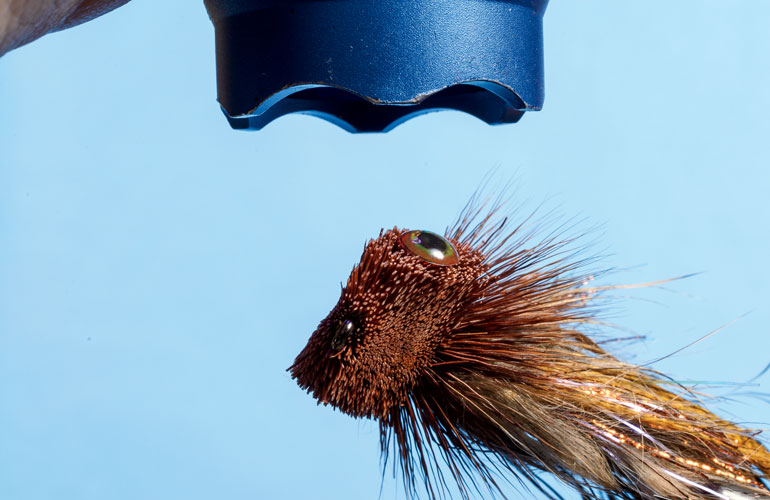The image is a close-up, full-color photograph of a detailed, intricately designed fishing fly lure, set against a light blue background. The lure itself is shaped like a small brown bug or sea creature, featuring a mixture of darker and lighter brown fur or hair protruding in various directions, giving it a wild, porcupine-like appearance. Prominently visible is a single, detailed eyeball on the right side of the lure, adding to its lifelike quality. At the top of the lure, there's a blue metallic component with curved ridges around the edge. This metal piece may be part of the mechanism for attaching the fishing line or for shaping the lure itself. The photograph is closely cropped, focusing on the intricate details of the lure, making the hook, if present, not visible.